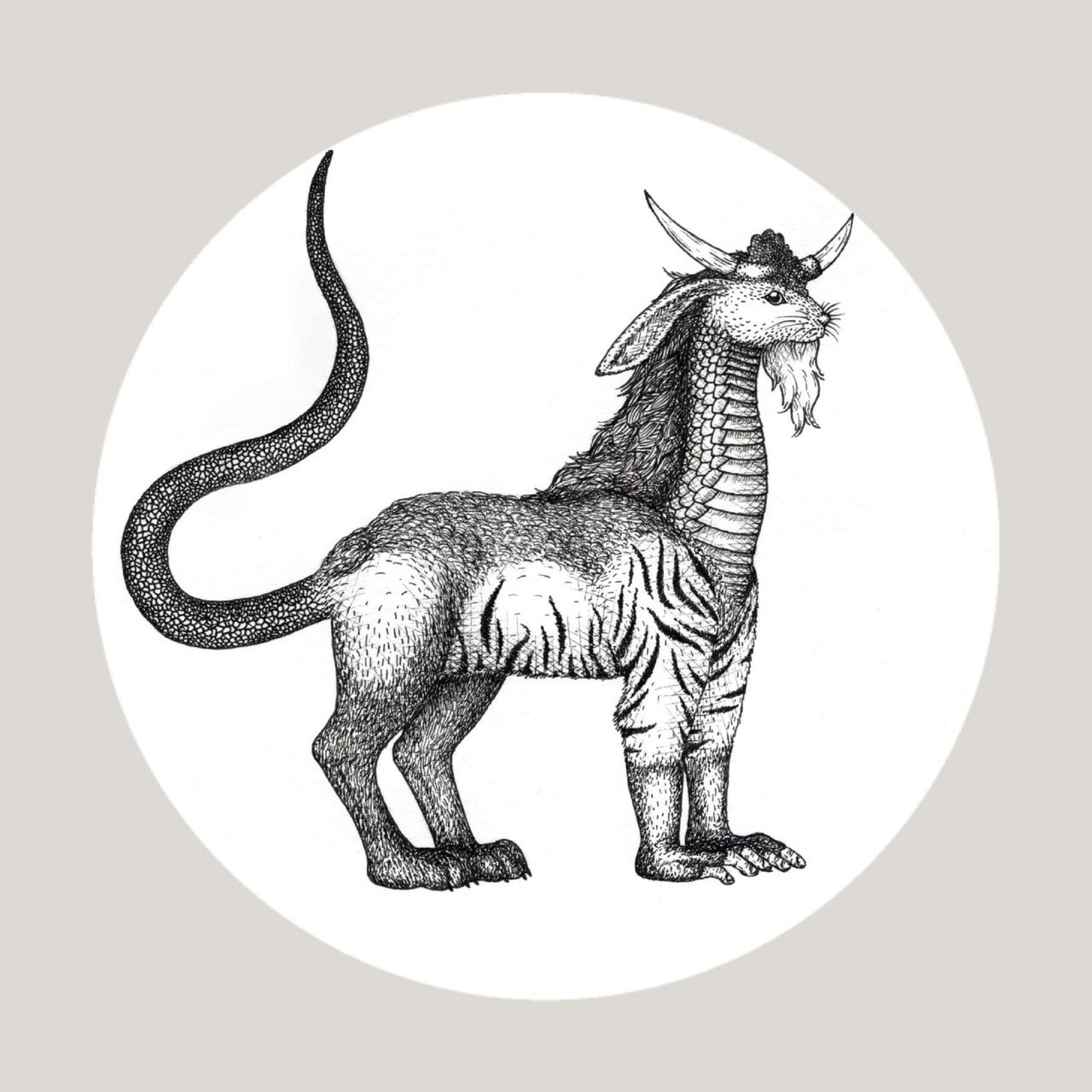The image features a detailed black and white drawing of a fantastical, hybrid creature encapsulated within a large white circle, set against a gray background. This unique being possesses characteristics from various animals, creating an intriguing, mythical appearance. 

From the left, the creature's long tail, resembling an octopus tentacle or perhaps a snake's, curls upward and occupies a significant portion of the white circle. The body transitions into furry hindquarters akin to those of a rabbit, while the back legs and paws resemble those of a large cat or horse, adding to its strength and mystique.

The midsection reveals stripes reminiscent of a zebra, extending across the belly and the front legs. Interestingly, these striped front legs transition into detailed, human-like or ape-like hands, showcasing a mix of strength and dexterity. Moving upward, the creature's elongated neck is covered in dragon-like scales, adding a reptilian element to its form.

At the top, the head is distinctly rabbit-like, complete with long, floppy ears and prominent whiskers. However, the creature also boasts bull-like horns protruding from its head, intertwined with tufts of hair. The face, with mouse-like features, further enhances the mythical essence of the illustration, combining elements from a wide variety of creatures into one seamless and captivating image.